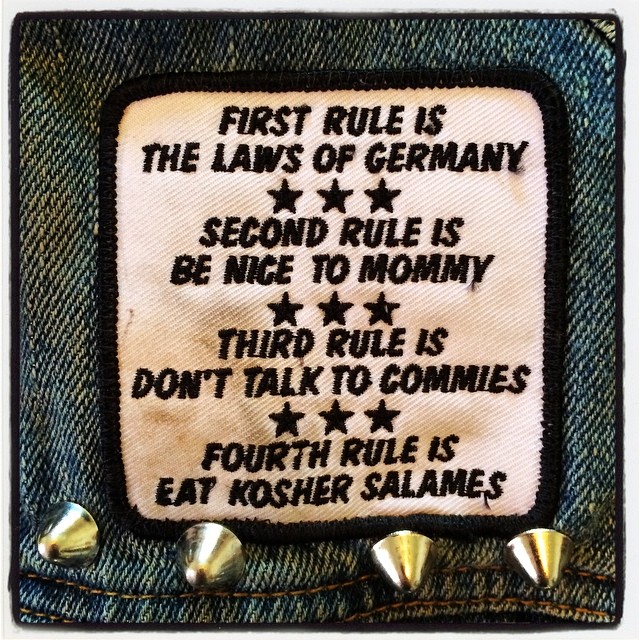This image features a detailed close-up of a punk-style denim jacket or vest, showcasing an embroidered patch prominently sewn onto a blue jean fabric. The patch has a light brown to white background with black text and a black border. It humorously lists four rules: "First rule is the laws of Germany," followed by three stars; "Second rule is be nice to mommy," also followed by three stars; "Third rule is don't talk to commies," accompanied by three stars; and "Fourth rule is eat kosher salamis," again with three stars. Below the patch, there are four metallic, pointed rivets or spikes, adding to the jacket's punk aesthetic. The stitching on the jeans is a contrasting yellow, and the fabric appears worn and slightly dirty, notably in the upper left and bottom right corners. The entire scene is captured in a photograph, emphasizing the patch as its central focus.